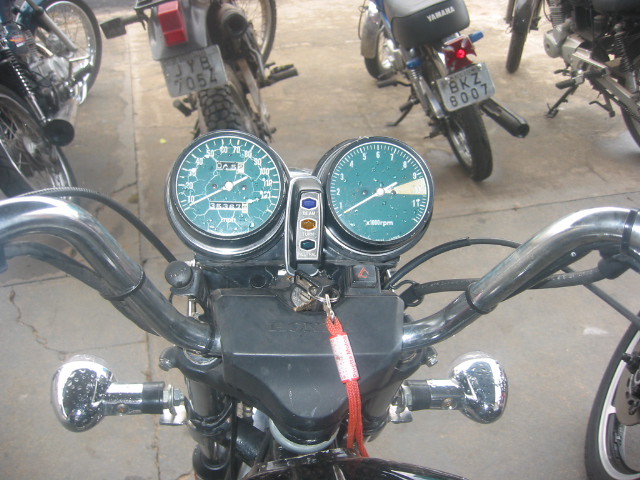The image presents a meticulous point-of-view shot from the perspective of someone seated on a motorcycle, gazing down at the dashboard. The motorcycle, reminiscent of a Harley-Davidson, showcases long, elevated silver handlebars that frame the scene. At the bottom center of the dashboard, a rectangular black section houses an ignition with a key plugged in. A vibrant red yarn keychain dangles from the keys, adding a pop of color.

Above the ignition, two bluish-green circular gauges dominate the view. The right gauge appears to be a tachometer, detailed with numbers ranging from 1 to 11 and a prominent white needle. The left gauge is identified as a speedometer, displaying various speeds in miles per hour. Small rectangular black windows on this gauge likely indicate the trip's total mileage.

Positioned centrally between the two main gauges, a vertical silver panel features three lights—blue, yellow, and dark green—presumably indicators for different functions of the motorcycle.

In the background, the scene extends to reveal the rear view of several smaller, narrower motorcycles lined up ahead. These motorcycles display visible license plates, seats, and back tires, adding depth and context to the primary view. The overall composition encapsulates the essence of a motorcycle convoy, poised and ready for the ride ahead.